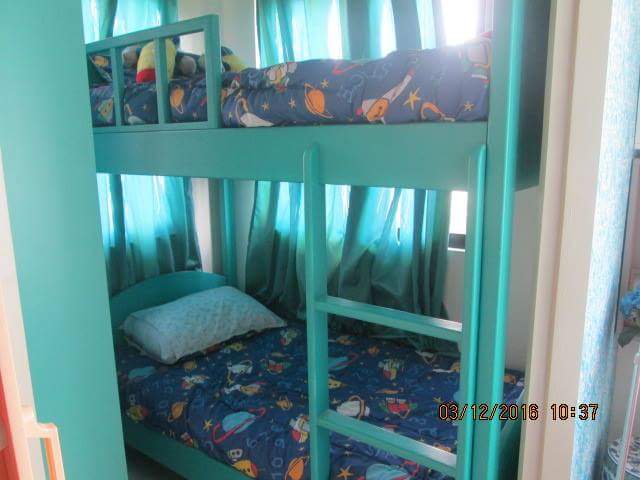This photograph captures a cozy child's bedroom featuring a vibrant light blue bunk bed with a playful space theme. The sturdy wooden frame, painted in a turquoise blue color, includes a matching ladder positioned on the bottom right, providing access to the top bunk. Both bunks are adorned with dark blue comforters decorated with cartoonish celestial patterns, including planets in shades of blue, orange, and white, along with colorful stars, spaceships, and astronauts.

The bedroom layout shows a white wall to the right side of the frame, contrasting with the turquoise blue wall on the left. Amidst the white wall to the right, a window with coordinating blue curtains lets in natural light, suggesting the photo was taken during daylight hours. Additionally, the background reveals a second window draped in similar blue curtains, enhancing the room's color scheme.

A date and time stamp reading "03-12-2016, 10:37" is visible on the bottom right corner of the image, confirming the photograph's capture date. The bottom bunk features two pillows—one blue and one with a white pillowcase—while the top bunk is decorated with stuffed animals, adding a touch of warmth and character to the scene. The arrangement of elements, from the cheerful bedding to the thoughtfully coordinated decor, creates an inviting and whimsical space for a child to sleep and dream.